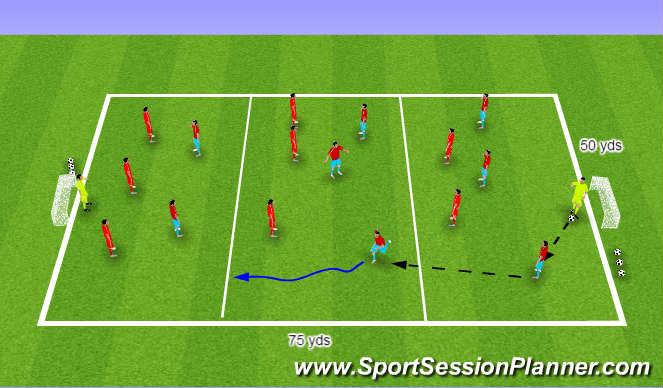The image is a horizontal rectangular screenshot from a digital soccer game or strategy session planner, specifically from the website www.sportssessionplanner.com, which is marked at the bottom of the image. The scene portrays a green soccer field, distinctly marked with white boundary lines and labeled dimensions of 75 yards in the middle bottom and 50 yards at the right end. The field features two goals, one at each end, with each goalie dressed in yellow.

Players are positioned across the field, viewed from a top-down perspective; some are in all red, while others wear red tops and blue bottoms. Arrows and lines indicate ball movement and strategies: a dotted black arrow shows the ball being kicked by the goalie on the right towards the left side of the field, aiming for midfield. A purple wavy arrow suggests further movement down the left side of the field. Additionally, the top of the image includes a light purple stripe running horizontally across. The overall layout and various on-field indicators emphasize a strategy planning scenario for a soccer match.